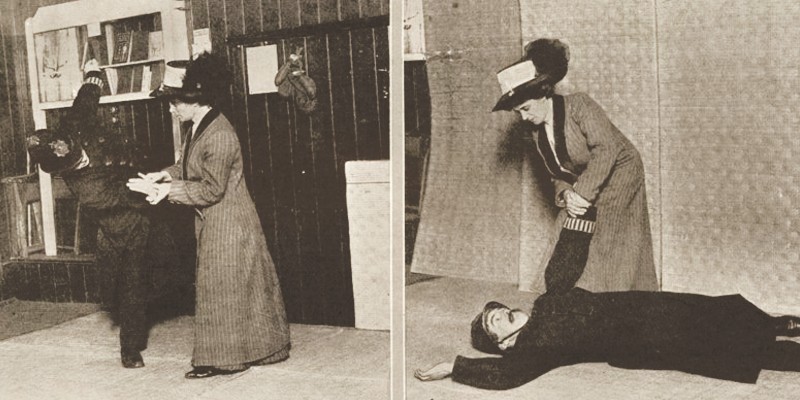This image is a horizontal two-panel composition with a light gray band dividing the black-and-white, sepia-toned photographs. Likely taken in the 1920s or 1930s, the pictures depict a dramatic scene involving a woman and a police officer in vintage attire.

In the left photograph, a woman in a long, striped dress and a black hat adorned with black feathers and a white bandana is standing. She appears concerned as she holds the hand of a police officer who is stumbling to his left. The officer, who has dark hair and a dark mustache, is dressed in a long black coat with brass buttons and a police hat featuring a small badge. Behind them, a bookshelf and a wooden wall can be faintly seen, adding context to the setting.

In the right photograph, the scene has escalated: the officer is now lying on his back on the ground, seemingly motionless, with his right hand outstretched above his head. The same woman stands above him, still holding his hand as if attempting to help him up.

The combination of these two striking images, complete with period-appropriate clothing and setting, creates a compelling narrative suggestive of a moment captured from an old-fashioned movie.